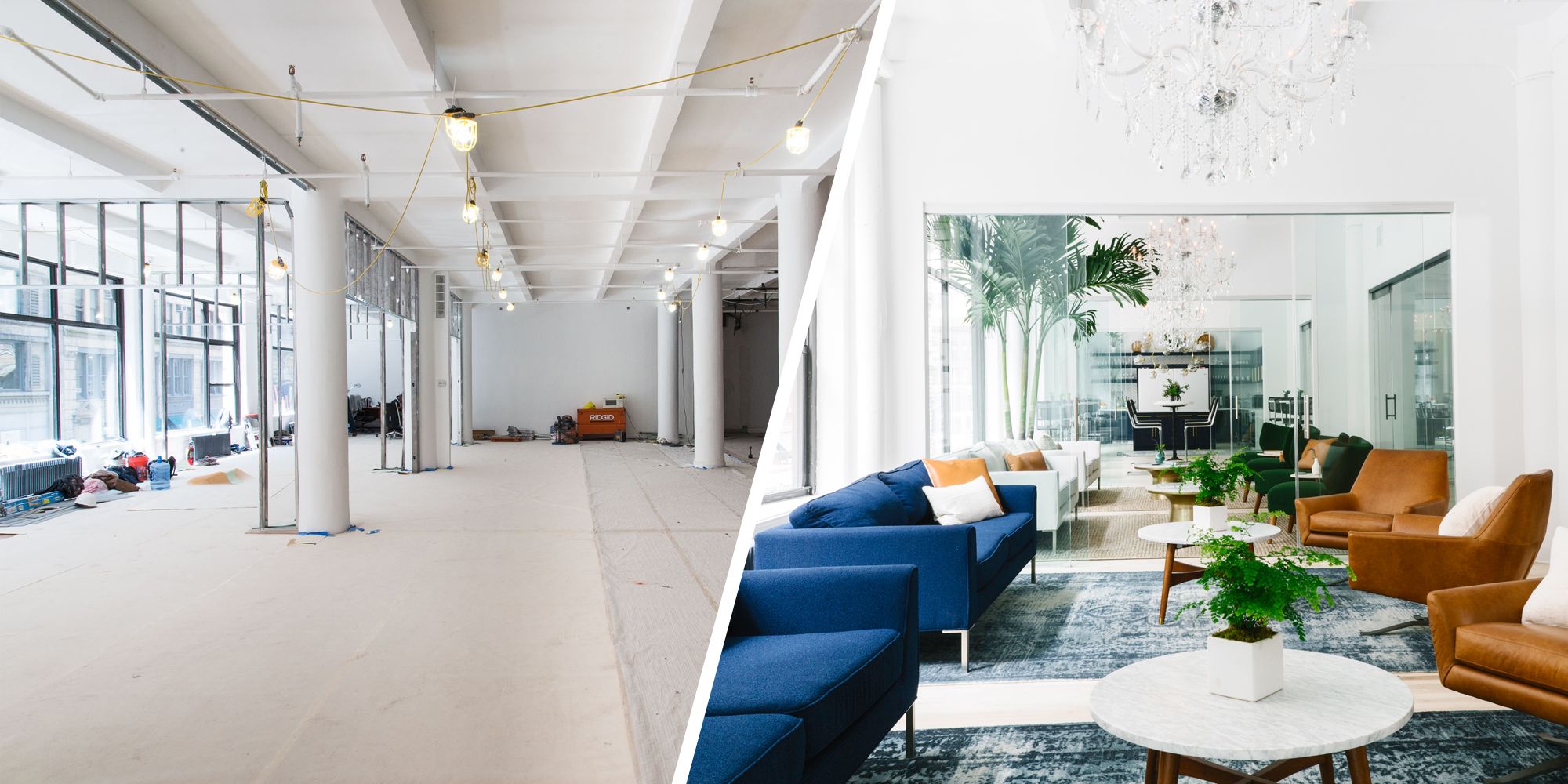The split image depicts the transformation of an office space from a construction site to a fully furnished and decorated room. The "before" photo on the left shows a spacious, white, and bare office with pillars lining the middle. Construction lights are strung across the ceiling with yellow cords, and various tools and cleaning supplies clutter the floor. A wall of large windows lines the left side, providing ample natural light. The "after" photo on the right reveals the same office space, now fully furnished. The room is decorated with two blue rugs, two blue couches, two white couches, and a mix of brown and black chairs with cushions. White tables, each adorned with green potted plants, are strategically placed among the seating. The ceiling is now clean and unobstructed, and the presence of additional tables and desks in the background suggests the room is now a functional office or waiting area.